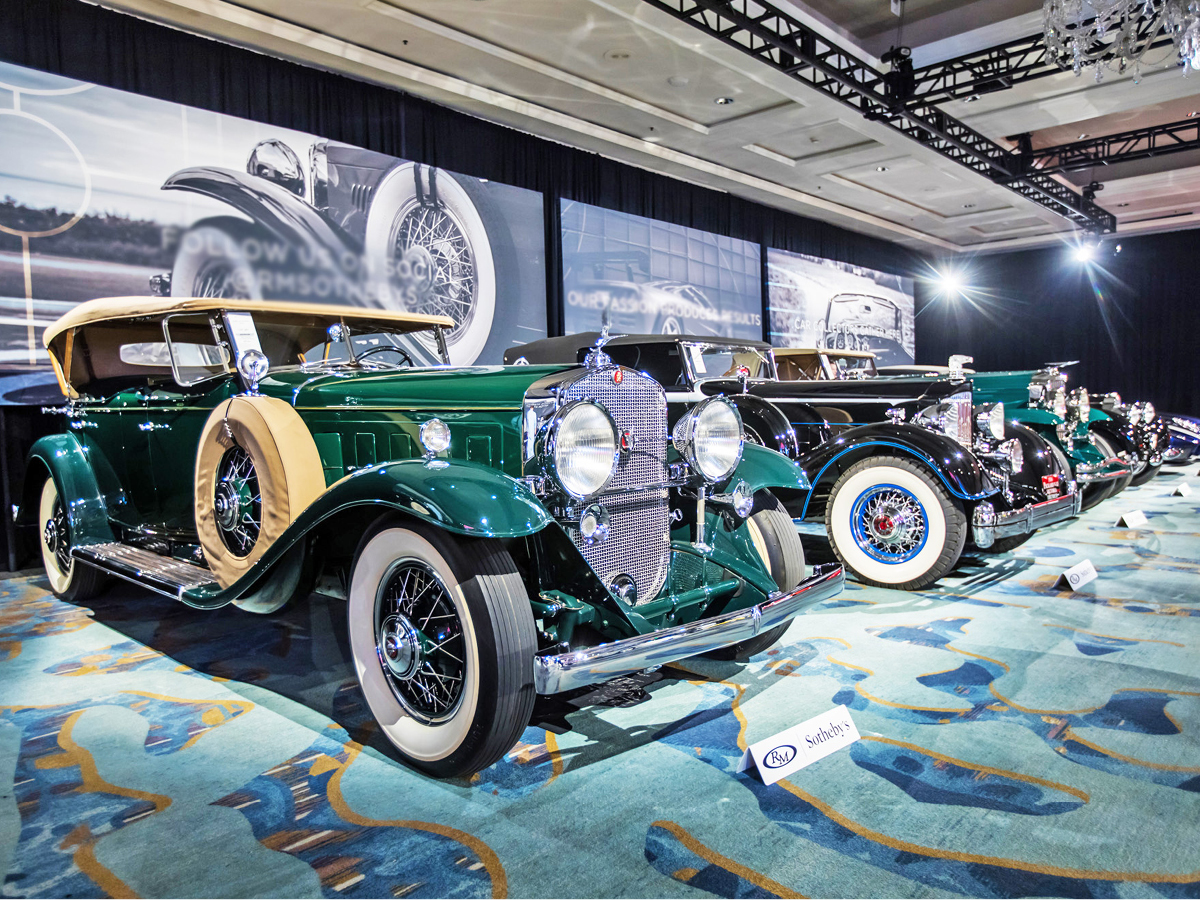The photograph captures a meticulously arranged showroom showcasing a stunning line-up of antique vintage cars, all in pristine condition. The cars are displayed against a backdrop of black and white photographs of similar classic automobiles, and the ceiling above is adorned with lights and black metal bars. The showroom floor features a decorative abstract carpet with hues of teal, blue, and gold.

Starting from the left, the first car is a striking green vehicle with a soft yellowish-beige roof and a matching spare tire cover. It boasts round headlights, curvy fenders, running boards, and whitewall tires, completing its vintage look. To its right, a black car with blue trim and blue rims stands in perfect symmetry, also featuring whitewall tires. Farther to the right, another green car with a white convertible top is visible, with additional vehicles, possibly black, extending further out of the frame.

Above these vehicles, the back wall displays a sign that reads "Follow us on social, @rmsotherbies" alongside a floor sign that says "R.M. Sotheby." This remarkable collection is set up in a museum-like ambiance, allowing visitors to admire these historic automotive treasures.